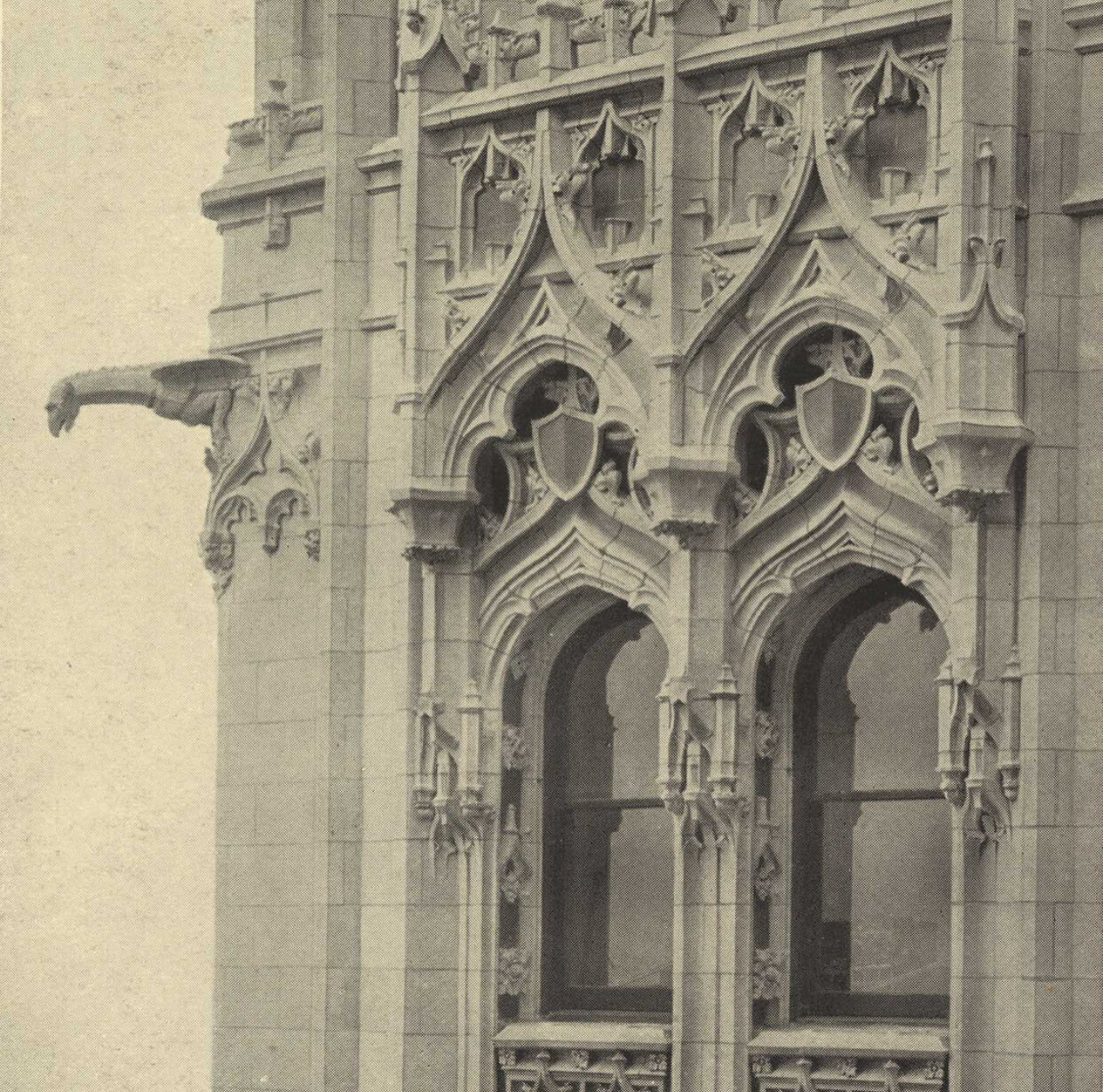The image depicts a sepia-toned, detailed photograph of the façade of a gothic-style church known as Skyrise Church. The upper portion of the building is shown, rendered in shades of light gray to dark gray, reminiscent of an old newspaper print or an aged photograph. The architecture is characterized by two prominent, vertically aligned windows with Romanesque arches at the top, each adorned with decorative shields. Above the left window, a gargoyle is perched, appearing to peer down from the side of the building. The building, which does not touch the ground nor show its top, dominates nearly 90% of the image, giving a sense of its towering presence. The entire scene evokes the architectural beauty and historical ambiance typical of structures from the 1300s to 1600s.